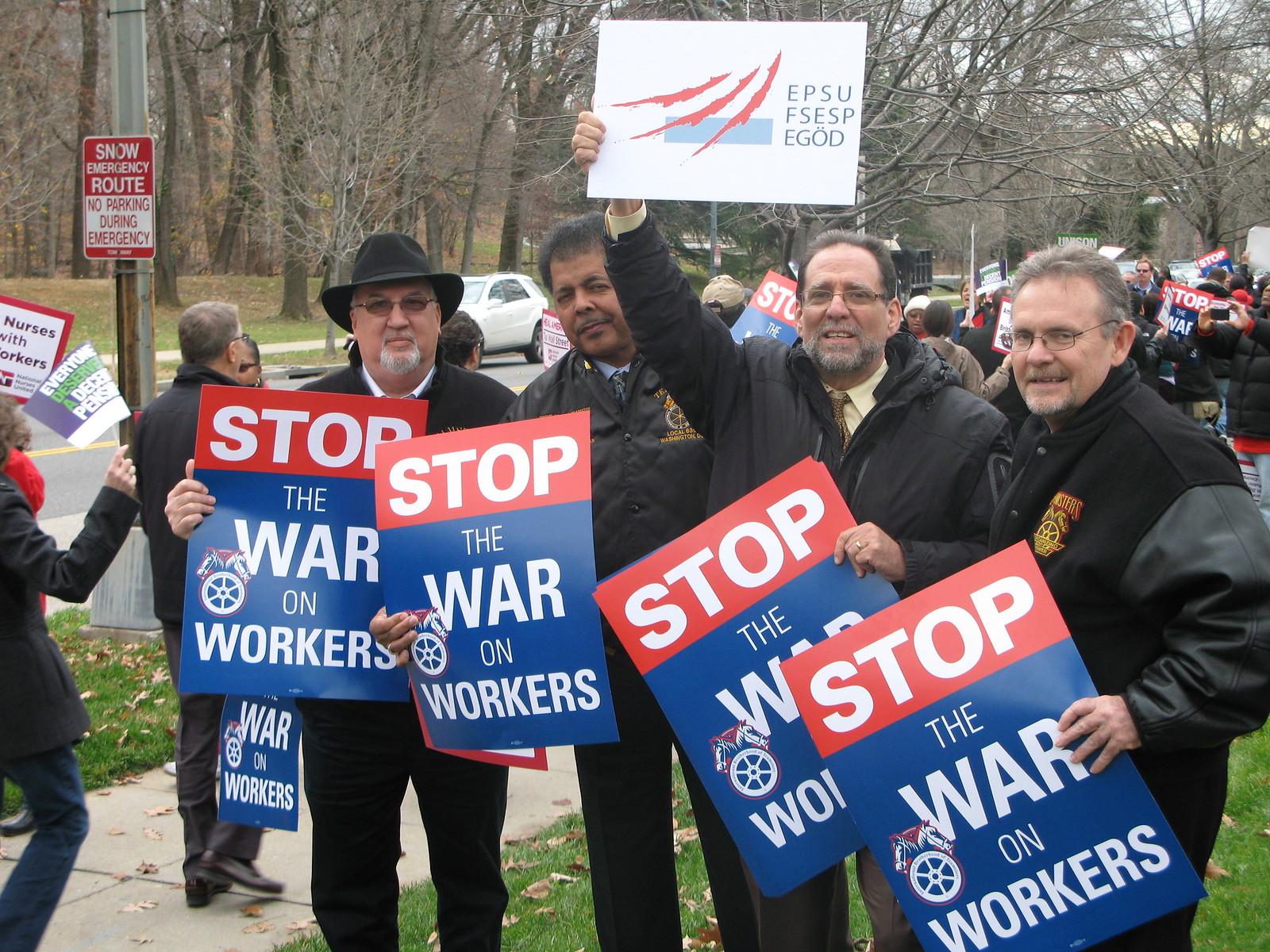The image captures a large protest scene during fall, indicated by the bare-branched trees in the background. At the forefront, four men in black coats stand prominently on a sidewalk and grassy area, each holding an identical sign with a red top and blue bottom. The top of the sign, in large white letters, reads "STOP," while the bottom states "THE WAR ON WORKERS." These men appear coordinated, with gold writing and a logo on their left chest pockets, suggesting possible affiliation to a particular organization. The second man from the left also holds an additional white sign with the acronyms "EPSU," "FSESP," and "EGOD," adorned with three curved lines over a horizontal blue rectangle. Behind them, a sizable crowd of 20-30 people also bearing signs can be seen, along with parked cars. The partly cloudy sky, visible in the upper right-hand corner, enhances the autumnal atmosphere of the protest for workers' rights.